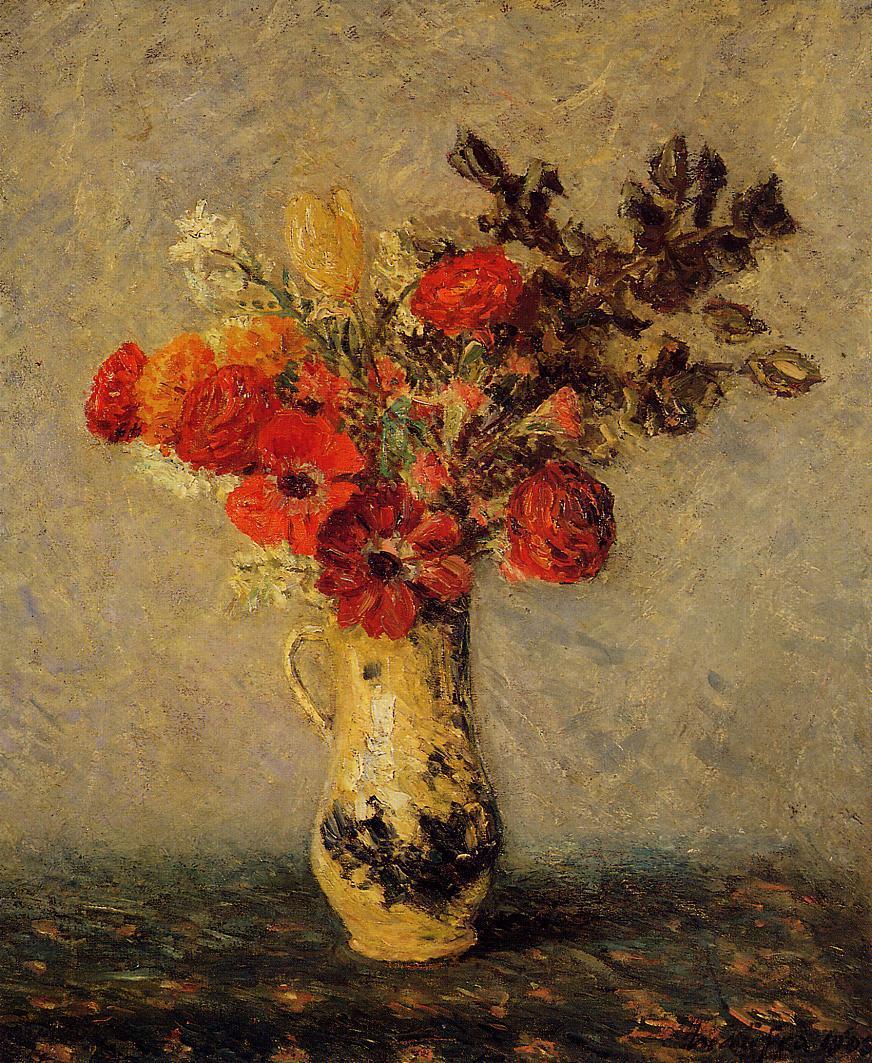The oil painting depicts a vase prominently placed on a dark brown table, set against a backdrop of grayish-beige and gold splotched walls. The vase itself is a golden mustard yellow with brown texturing, adding depth and harmonizing it with the table. It features a handle extending to the left, enhancing its classical appearance. The vase is brimming with a diverse array of flowers, predominantly in shades of red and orange, with some branches and foliage, including dark brown leaves. The assortment includes recognizable blooms such as lilies, roses, petunias, anemones, and ranunculus, with splashes of pink, white, and gold among them. Some white flowers appear to be on stalks, adding to the dimensionality of the arrangement. The image is vibrant, with colors like yellow, black, white, brown, pink, orange, red, green, and off-white intermingling. A tiny, indecipherable text scrawl is present at the bottom right corner of the painting.